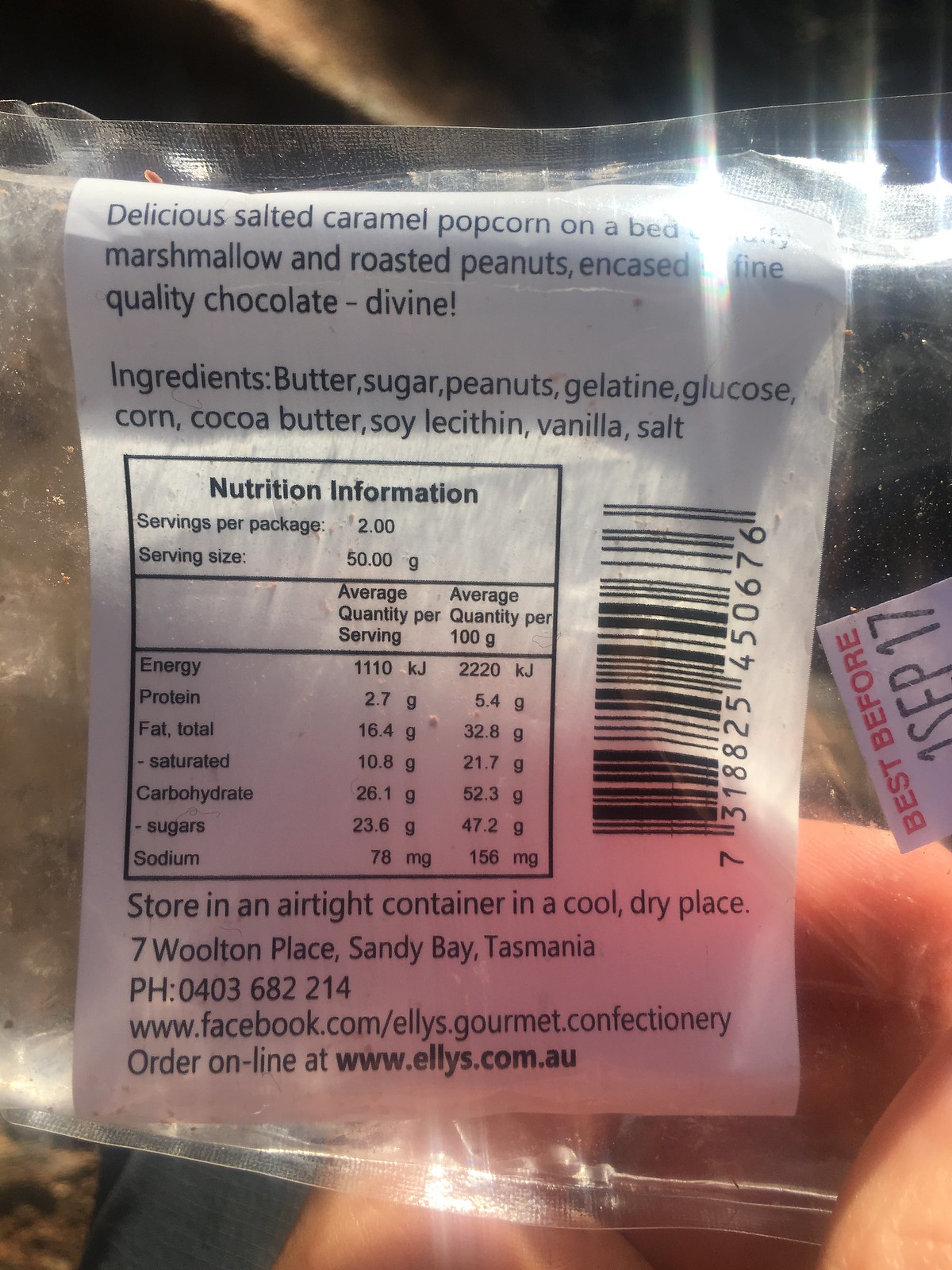In the image, we see a close-up of a white plastic package that once contained snacks. It's being held by a person with fair skin. The photo appears to have been taken outdoors at night, with the dark, black sky in the background providing a stark contrast to the package. The package itself is clear and square, now empty but showing signs of smeared remnants from the delicious treats it held. The white label on the back of the package reads, "Delicious Salted Caramel Popcorn on a Bed of Marshmallow and Roasted Peanuts encased in fine quality chocolate, divine." Additionally, the label lists the ingredients: butter, sugar, peanuts, gelatin, glucose, corn, cocoa butter, soy lecithin, vanilla, and salt, along with some nutritional information. The messy state of the package indicates that the snacks inside were thoroughly enjoyed.